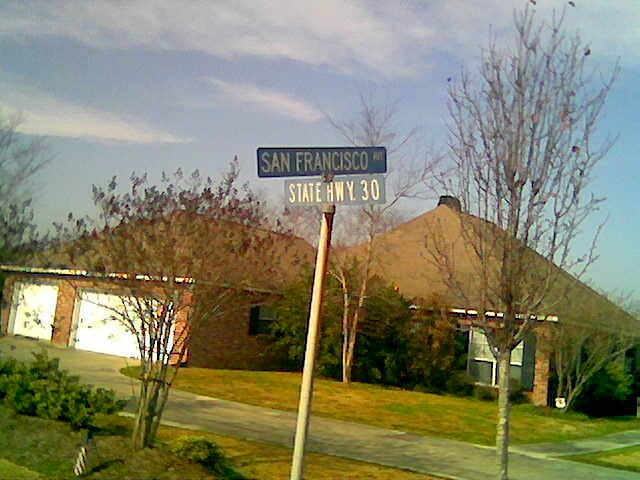In this photograph, a charming brick single-story home is prominently displayed in the center of a residential neighborhood. The house features an attached two-car garage and sits amidst a verdant yet slightly brownish lawn, indicative of recent weather changes. Surrounding the home, several young trees suggest recent landscaping efforts to enhance the greenery. 

The paved driveway extends from the street to the garage, providing a clean and accessible entry point to the property. Above the home, the sky stretches wide, painted a serene shade of blue interspersed with white, wispy clouds that add texture and depth to the scene.

A notable detail in the foreground is a street sign mounted on a metal pole, prominently marking the intersection with green rectangular signs. The white lettering clearly designates this locale as the junction of San Francisco Avenue and State Highway 30, providing useful context and direction for onlookers and visitors alike. This idyllic suburban setting captures the essence of comfortable residential living, framed by natural and structural elements in perfect harmony.